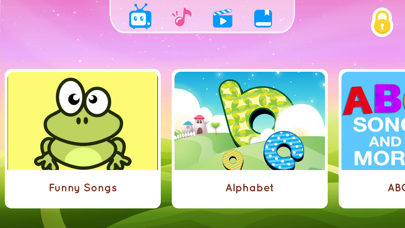Against a bright pink background, the top section features a series of colorful icons inside a pink rectangle. Starting from the left, there is an image of a blue television with blue antennas. The TV screen is white, with two blue circles resembling eyes. 

To the right of the television, there's a pink musical note, followed by a clapperboard icon used by directors to signal the start of a scene. The clapperboard is square-shaped with a white arrow in the middle, blue and white stripes at the top, and mainly blue and white colors.

Further to the right is a yellow lock symbol. Below these icons, there is a yellow square featuring an animated green frog with whimsical, mismatched eyes—the left eye being notably larger than the right. Beneath the frog, the text reads "Funny Songs."

Adjacent to this, large letters "A," "B," and "C" are prominently displayed against a backdrop of a blue sky with clouds. Below the letters, the word "Alphabet" is written. To the far right, the background is blue featuring the letters "A" in red, "B" in purple, and the phrase "Songs and More."